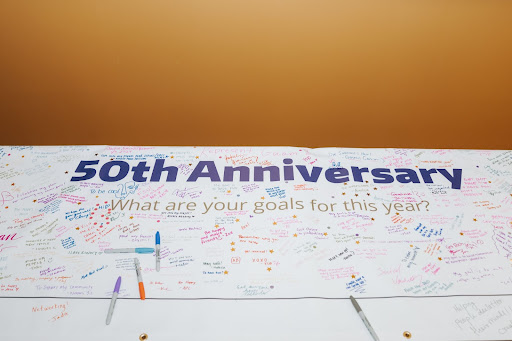This photograph captures a white banner celebrating a 50th Anniversary, prominently displayed against a burnt orange backdrop. The banner features large blue letters proclaiming "50th Anniversary," with smaller gold text beneath that reads, "What are your goals for this year?" Scattered across the banner are an array of colorful Sharpies—purple, blue, orange, and silver—indicating that participants have used them to write their goals. The banner is densely covered with multicolored messages and signatures in various sizes and directions, suggesting the involvement of upwards of 100 people. Two brass eyelets at the bottom of the banner hint at it being hung for display. The image captures the essence of a communal celebration, with the banner serving as a vibrant testament to collective aspirations and milestones.